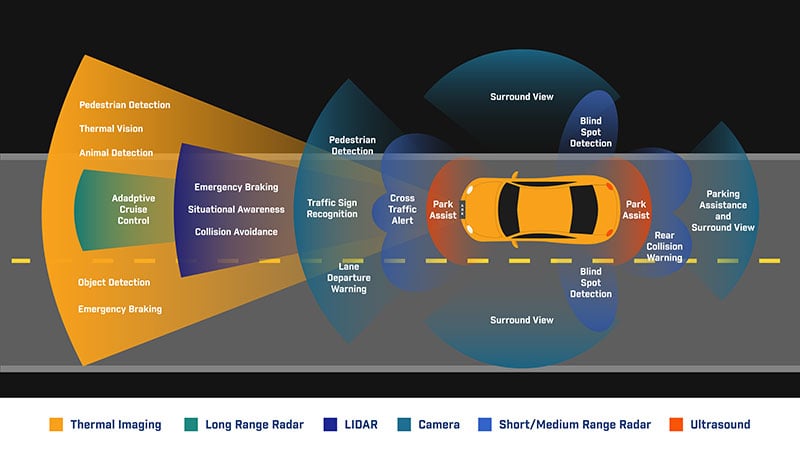The image depicts a detailed, animated diagram of a yellow vehicle with black windows driving on a road marked by a central yellow line and black sides. Surrounding the car are various colored bubbles, each indicating different advanced vehicle functions and detection features, such as pedestrian detection, thermal vision, animal detection, adaptive cruise control, object detection, emergency braking, situational awareness, collision avoidance, traffic sign recognition, lane departure warning, cross traffic alert, park assist, surround view, blind spot detection, and rear collision warning. The car is part of a computer simulation showcasing its high-tech safety and assistance systems. Each function is color-coded based on a legend at the bottom: gold for thermal imaging, green for long range radar, dark blue for lidar, teal for camera, blue for short and medium range radar, and orange for ultrasound. This comprehensive portrayal offers a clear view of the car's capabilities and the technologies employed to ensure a safe driving experience.